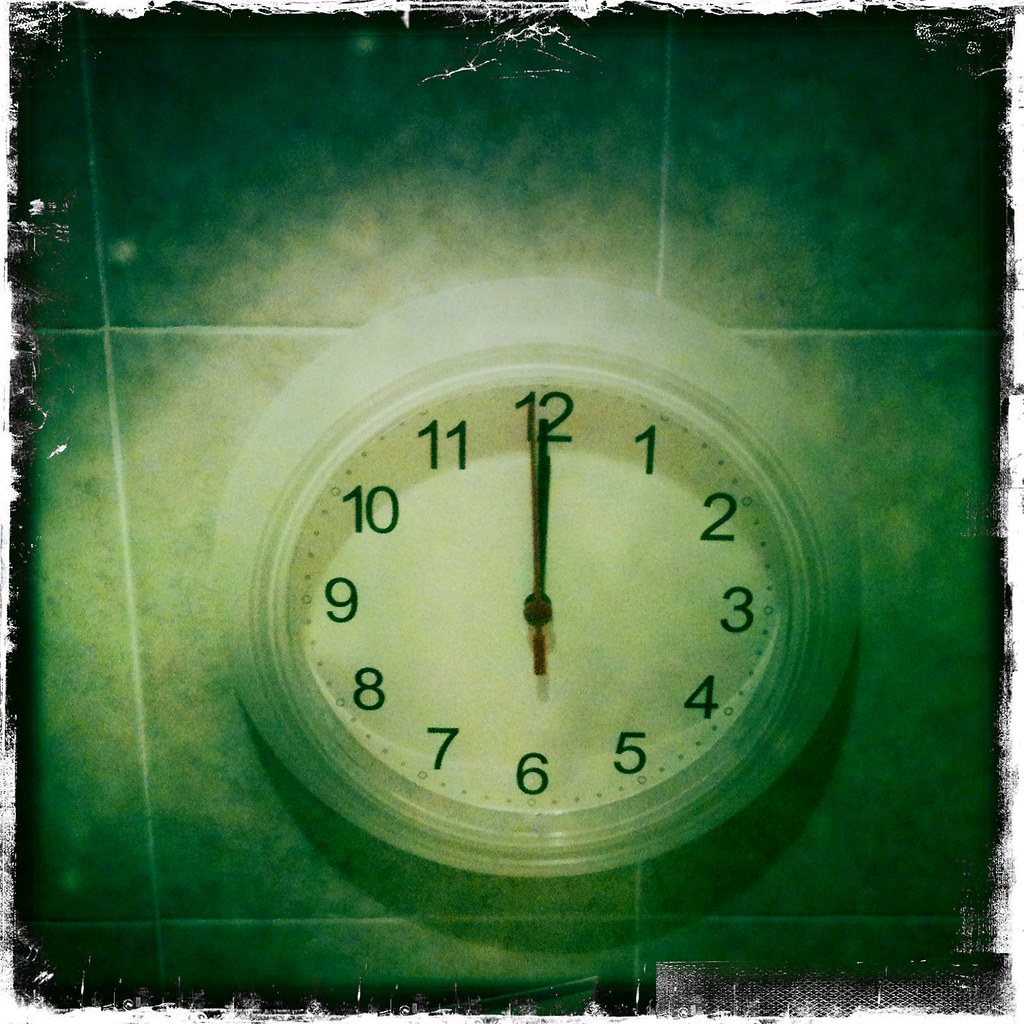This image depicts a clock situated against a green-tiled background, rendered in a highly artistic and evocative manner. The clock itself is vividly illuminated, with a bright white border and face, contrasting sharply against the splotchy black border that surrounds the entire scene. The numbers on the clock are boldly black, and the hands, also black, are pointed straight upward, indicating it is either noon or midnight. The artistic elements, including the irregular black splotches framing the image, evoke the feel of a comic book cover, an album cover, or an imaginative advertisement, giving the overall composition a striking and stylish appearance.